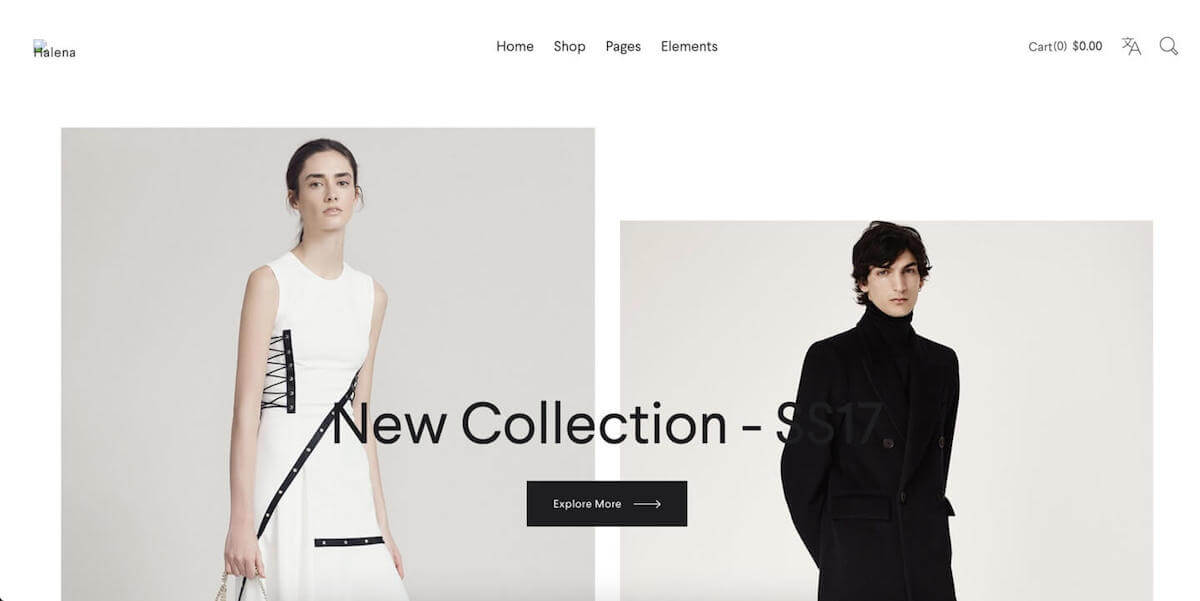A screenshot from a clothing website. At the top center, there is a navigation menu with the tabs: "Home," "Shop," "Pages," and "Elements." On the far right of the menu, there is a "Cart" section, which shows "0" items and a total of "$0.00." Next to this, there is an icon that appears to be for language translation. In the main section of the screenshot, two images are prominently displayed. The image on the left features a woman wearing a white dress, while the image on the right showcases a man wearing a black shirt.